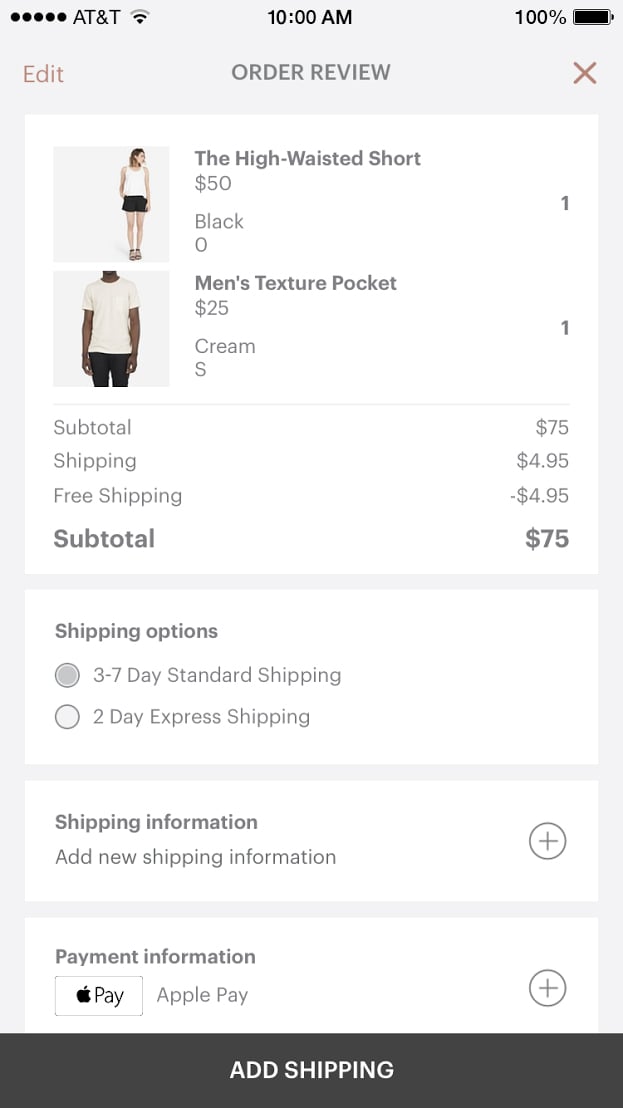The image appears to depict a slightly blurred printout of a digital shopping interface, likely from a mobile device using AT&T for internet at 10 a.m., with the device displaying a 100% battery level. 

At the top of the screen, there are navigational buttons that read "Edit" and "Order Review," with the "Edit" button highlighted in brown. Below, the page includes product images and descriptions:

1. A photo of a girl dressed in a white top paired with a blue or black skirt. The adjacent description reads: "High-Waisted Shorts, $50, Black, Quantity: 1".
2. An image of a person wearing a white short-sleeved t-shirt with black bottoms. The description to the right indicates: "Men's Texture Pocket T-shirt, $25, Cream, Quantity: 1".

Following the product descriptions is a section detailing the order summary:
- Subtotal: $75
- Shipping: $4.95
- Promotion: Free Shipping ($4.95 off)

Next, the section labeled "Shipping Options" outlines the chosen method of "3-7 Days Standard Shipping," with the alternative option being "2-Day Express Shipping."

Below, the "Shipping Information" section includes an option to "Add New Shipping Information." 

In the "Payment Information" section, the payment method selected appears to be Apple Pay, accompanied by the Apple Pay logo.

At the bottom, there's a button against a black banner with white text that reads "Add Shipping."